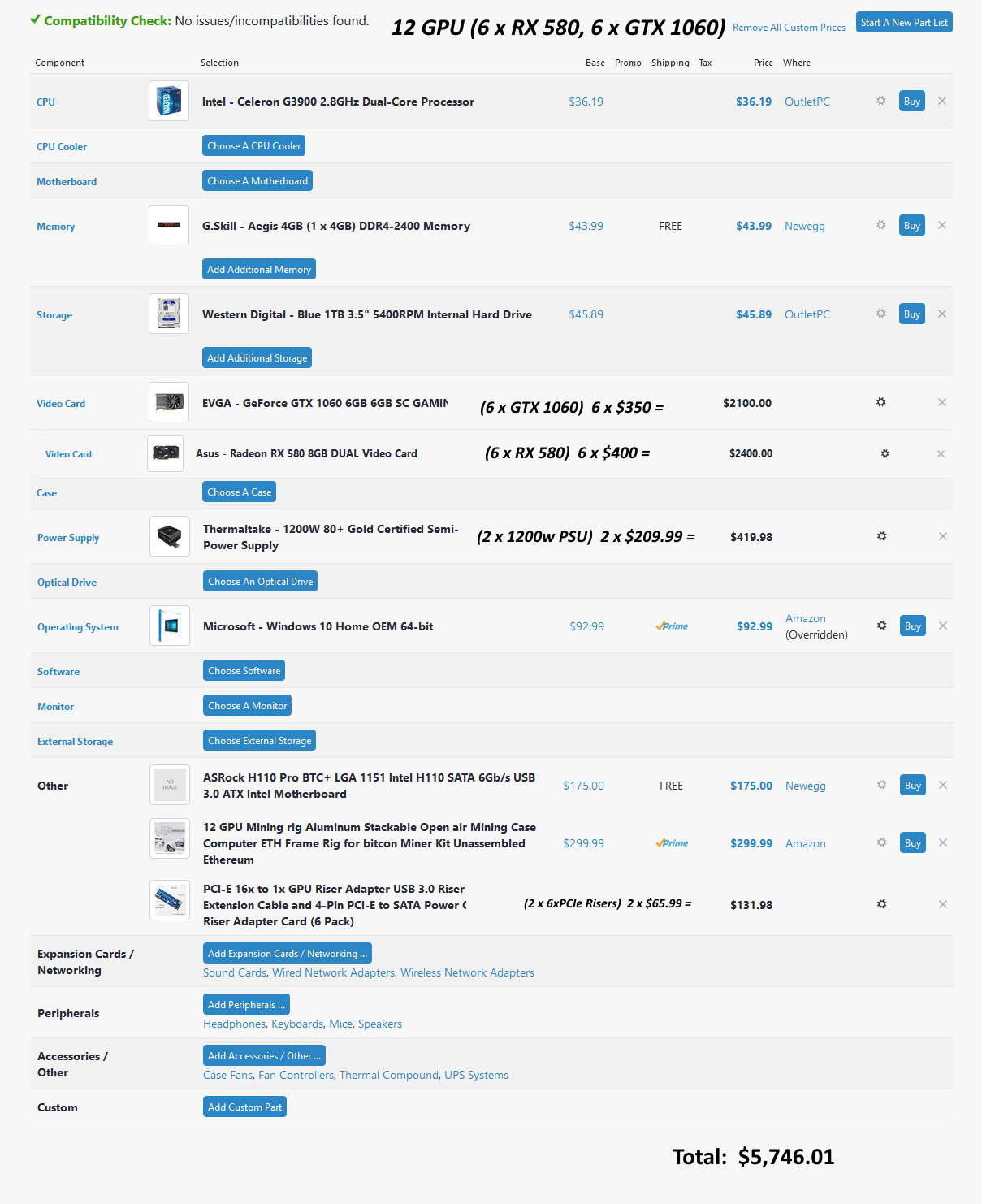This image displays a detailed breakdown of a PC checkout screen from a custom PC builder website, evidently set up for creating a cryptocurrency mining rig. At the top of the screen, a prominent green check mark is accompanied by a message stating "Compatibility check: no issues or incompatibilities found," ensuring that all selected components are compatible.

The main section of the screen highlights the inclusion of 12 GPUs, divided evenly between 6 RX 580s and 6 GTX 1060s. A new price list section follows, organized into multiple columns for component selection, base price, promotional price, shipping costs, tax, and the total price.

On the left side of the screen, a detailed list of components is displayed, including:
- CPU: Intel Celeron G3900 2.8 GHz Dual-Core Processor
- CPU Cooler
- Motherboard
- Memory (RAM)
- Storage (Hard Drives/SSDs)
- Primary Video Card: GeForce GTX 1060 6GB (6 units at $350 each, totaling $2,100)
- Secondary Video Card: Asus Radeon RX 580 (6 units, totaling $2,400)
- Case
- Power Supply
- Optical Drive
- Operating System
- Software
- Monitor
- External Storage

The screen also dedicates space for additional items such as:
- Expansion Cards
- Networking Options
- Peripherals
- Accessories
- Other Custom Components

At the bottom of the screen, the total cost for all selected items is prominently displayed, amounting to $5,746.01. Options are also available for selecting and adding more components to enhance the mining rig's capabilities. The combined price for just the GPUs alone is around $4,500, illustrating the significant investment in graphical power required for cryptocurrency mining.